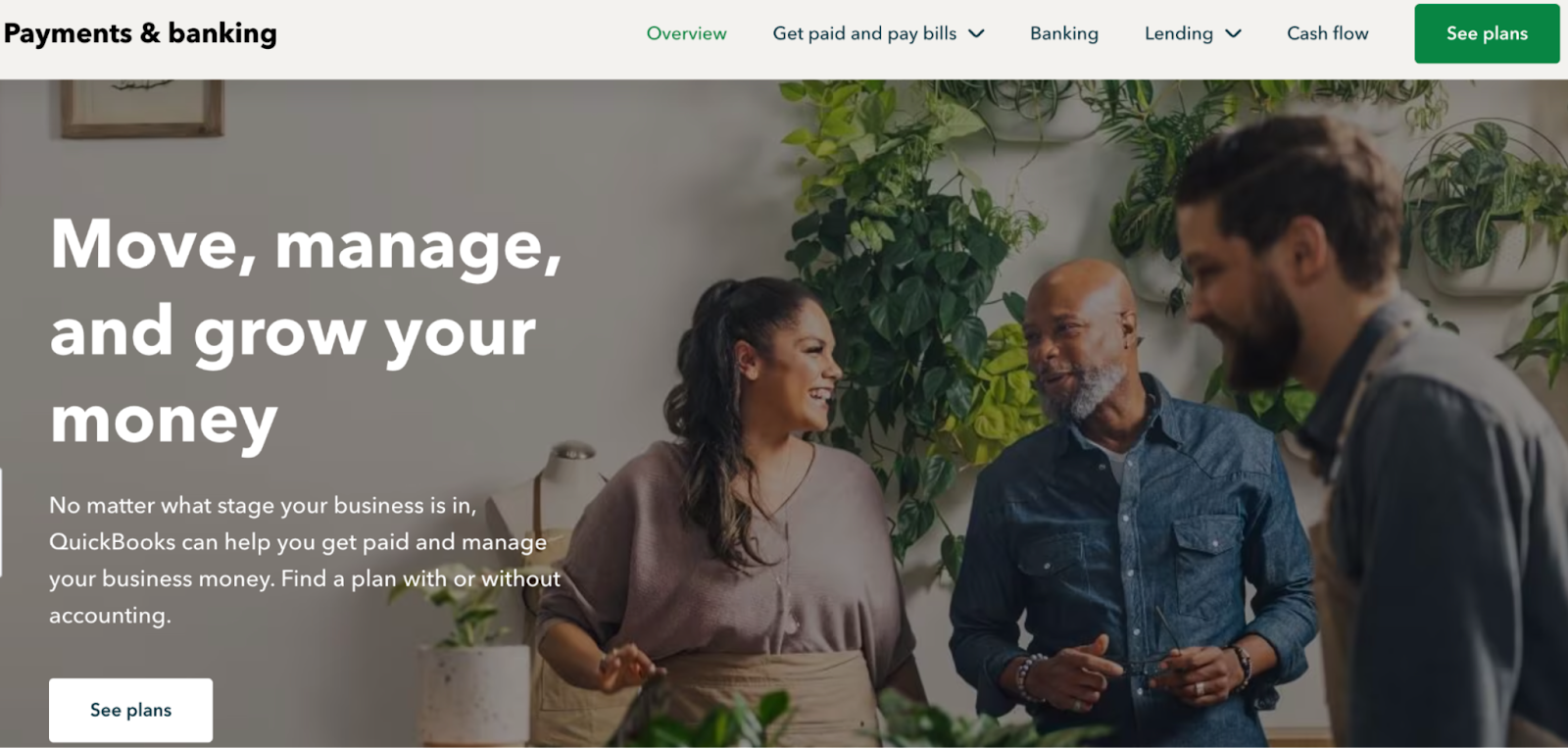The image depicts a section of a financial website designed to help users manage and grow their money. The website's interface is clean and straightforward, with a bold header that reads "Payments and Banking." Below this header, there are five navigational options: "Overview" (highlighted in green), "Get Paid and Pay Bills" (with a dropdown menu), "Lending" (with another dropdown menu), "Cash Flow," and "See Plans" (also highlighted in green). 

The central part of the image features a couple. The man, who has a bit of facial hair, is dressed in a button-up denim shirt, accessorized with a wristwatch, a wedding ring, and a bracelet. The woman, who has long hair and is smiling at the man, wears a beige dress. Behind them, plants adorn the wall, adding a touch of greenery to the scene. A third person, a man with a beard, is captured in a side shot walking in front of the couple. He is dressed in a long-sleeve shirt. 

Beneath this imagery, the website's tagline "Move, Manage, and Grow Your Money" is laid out across three lines, followed by a subheading that encourages users to sign up. There is a prominently displayed "See Plans" button in white. The website provides multiple options for users, including online bill payments for those who already have an account.